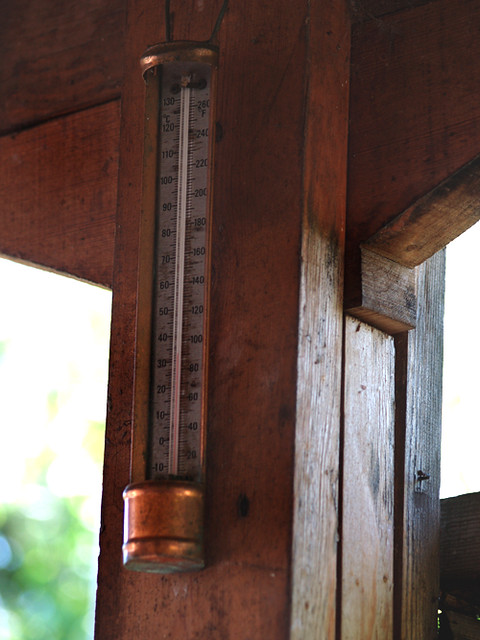This captivating image showcases an antique thermometer, encased in a thick, robust copper frame that exudes a sense of quality craftsmanship despite its evident age. The thermometer hangs from the upper rafters of an open wooden structure, characterized by dark-stained wood that reveals rich, varied grains and knots, adding to its rustic charm. The wooden pillar, square and four-sided, serves as a backdrop, with a gray sky visible through its gaps. To the left of the pillar, the silhouette of a tree adds a touch of natural beauty to the scene.

The thermometer, suspended quite high, features black numerals on a white background, with the red mercury line faintly visible just below 40 degrees, though its precise end point is unclear. The device is housed within a unique copper casing: at the top, a round decorative element, and below it, a thicker circular detail, both enhancing its antique appeal. A C-shaped column encloses the thermometer tube, completing the intricate design. The entire apparatus hangs from a black fixture, blending practicality with aesthetic allure.